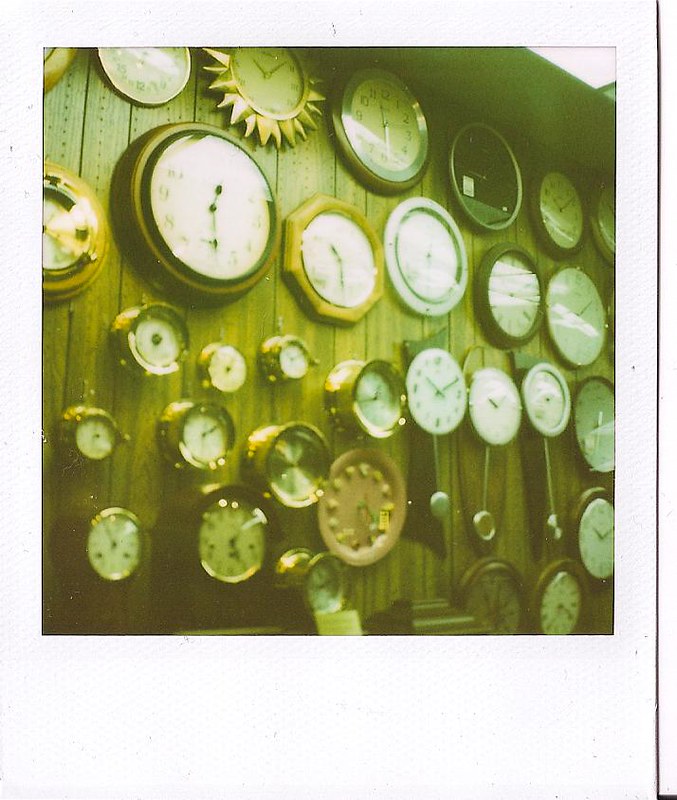The photograph displays a rustic dark brown wooden wall adorned with an eclectic collection of clocks, each set against the vertical grain of wooden planks. This assemblage features multiple rows of closely arranged timepieces, predominantly circular in shape, but interspersed with unique designs including star-shaped and octagonal clocks. Captured with a grainy texture that evokes a vintage aesthetic, the image exudes a nostalgic ambiance. Most clocks exhibit a classic white face with black numerals and hands, although a few boast elegant gold and metallic casings. The overall scene is slightly blurry, further enhancing its old-fashioned charm.